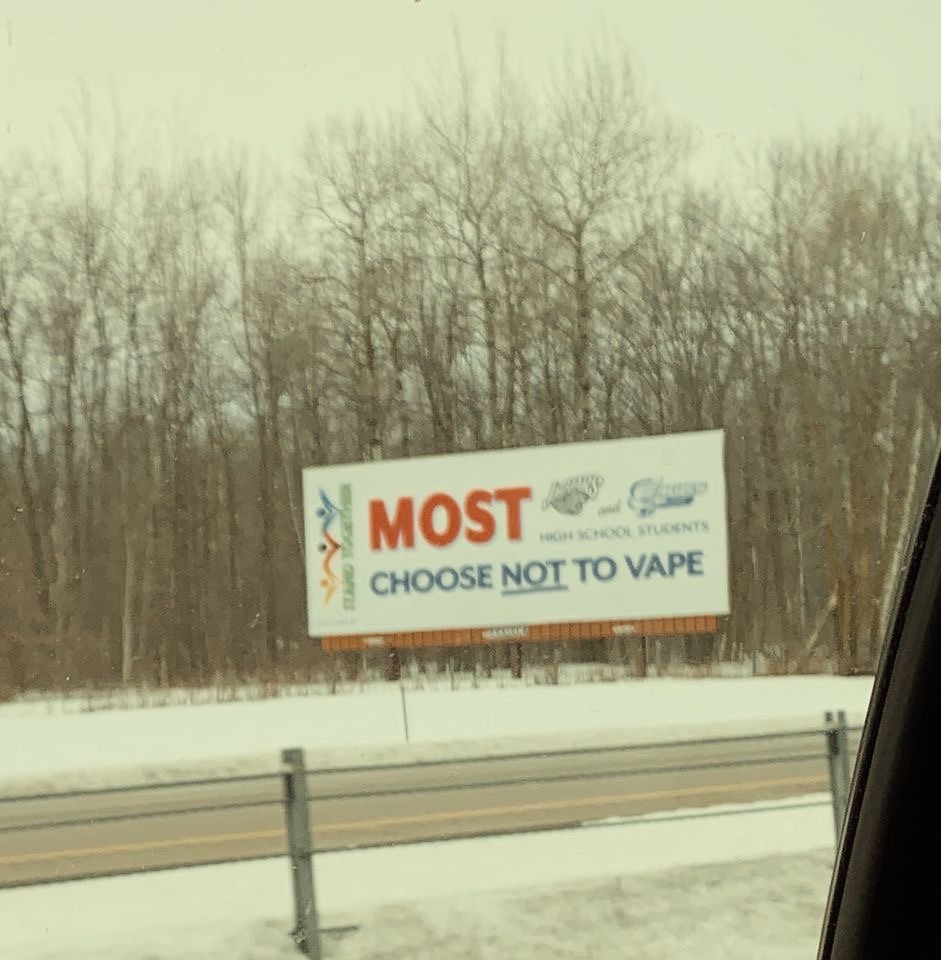A photograph captured in winter, devoid of any visible grass, reveals a bleak yet intricate landscape. The ground is entirely blanketed in snow, and the view seems to be from the inside of a car, probably through a window. On the edge of the frame, the outline of a car door is faintly visible. Beyond this, a typical interstate metal barrier fences off the road. In the background, a row of trees stands barren, stripped of their leaves by the cold season, contributing to the overall gloomy atmosphere. Dominating the scene is a large billboard with a pristine white background, prominently displaying the word "Most" in bold red letters. Below it, a smaller text reads, "High School Students Choose Not to Vape," accompanied by images of vape pens. The billboard is completed with a sponsor's logo, though the details of the logo remain indiscernible. The entire composition, set against a dull, overcast sky, creates a stark depiction of a winter day marked by muted yet compelling details.